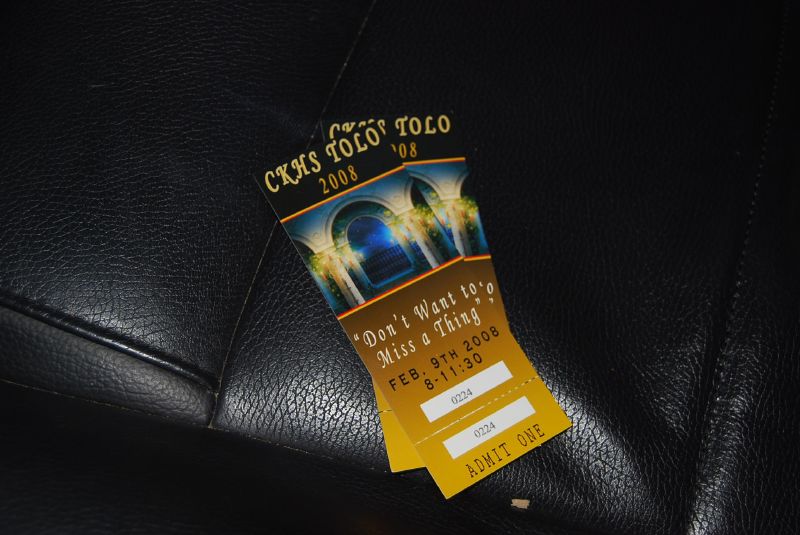The image is an overhead close-up of two identical tickets resting on a black leather seat, possibly from a car or a couch. Each ticket features the heading "CKHS Tolo 2008," followed by an illuminated archway that suggests a festive, castle-like entrance. Below the archway, in an orange section, the phrase "don't want to miss a thing" is quoted. The event details read "February 9th, 2008, 8-11:30," and each ticket bears the number 0224. There's a perforated strip where "0224 Admit One" is repeated, indicating an entry pass. The tickets are positioned one on top of the other, both prominently displayed against the shiny black leather surface.